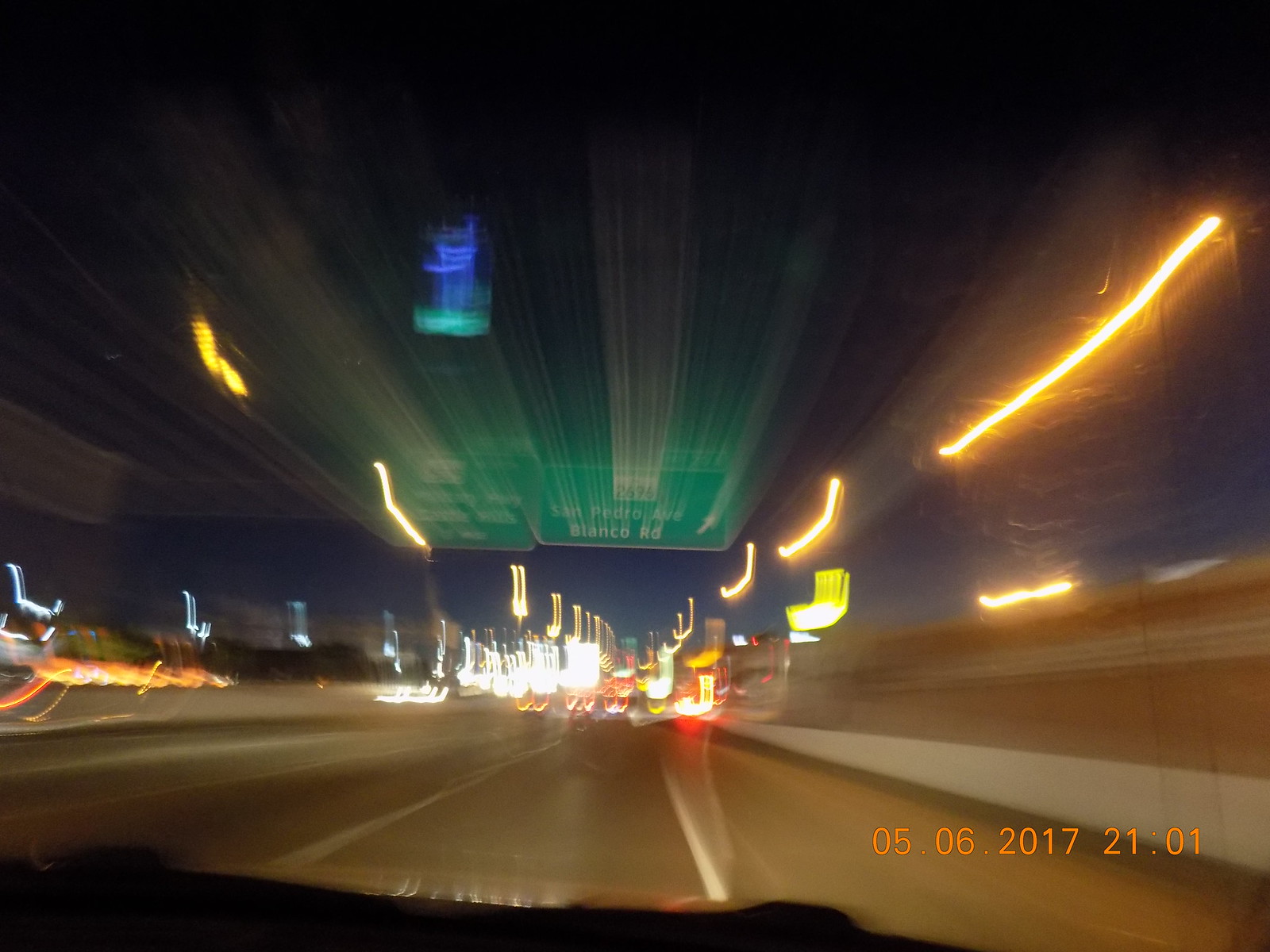The image captures a night-time scene taken from inside a moving vehicle, likely using a dashboard camera. The photograph is a still frame that shows a stretch of a highway or expressway. The road appears smooth and is flanked by walls on both sides, separating the lanes of traffic. There's a central divider demarcating the flow of vehicles traveling in opposite directions. 

The scene is enveloped in darkness, with several blurred lights indicative of distant taillights and headlights from other vehicles. The overall visibility is poor due to the blurriness of the image. Two green highway signs are partially visible, though they are also quite blurry. One of these signs bears the names "San Pedro Avenue" and "Blanco Road," though the text is difficult to discern clearly. Despite the lack of clarity, the photograph effectively conveys the sense of traveling on a nighttime highway, guided by the dim glow of traffic lights and the faint, familiar markers of road signs.